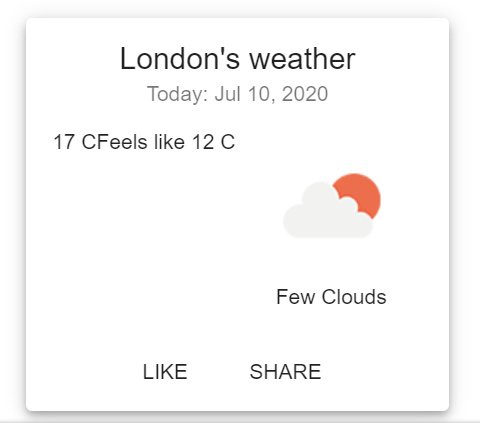The image features a square box set on a solid white background. At the top center of the box, bold text reads "London's Weather," indicating that the box displays weather information. Beneath this heading, in smaller, grayish text, is the phrase "Today: July 10th, 2020," providing the date.

In the upper part of the box, slightly to the left, the temperature is displayed as "17°C," followed by "Feels like 12°C." This segment details the current temperature and perceived temperature.

On the middle-left side of the box, there is an empty space, emphasizing the simplicity and clean layout of the design. The middle-right area contains a weather icon: a light gray cloud with an orange sun partially visible behind it, representing partly cloudy conditions. Directly below this icon is the label "Few clouds," describing the weather.

At the bottom of the box, to the left, the word "Like" is displayed, followed by an empty space and then the word "Share." These likely represent interactive options for social media engagement. The presence of two empty spaces on either side of these words suggests a balanced and minimalistic design choice.

Finally, a horizontal line spans the entire width of the image at the very bottom, outside the confines of the box, accompanied by a shading effect above it, adding a subtle visual boundary to the overall composition.